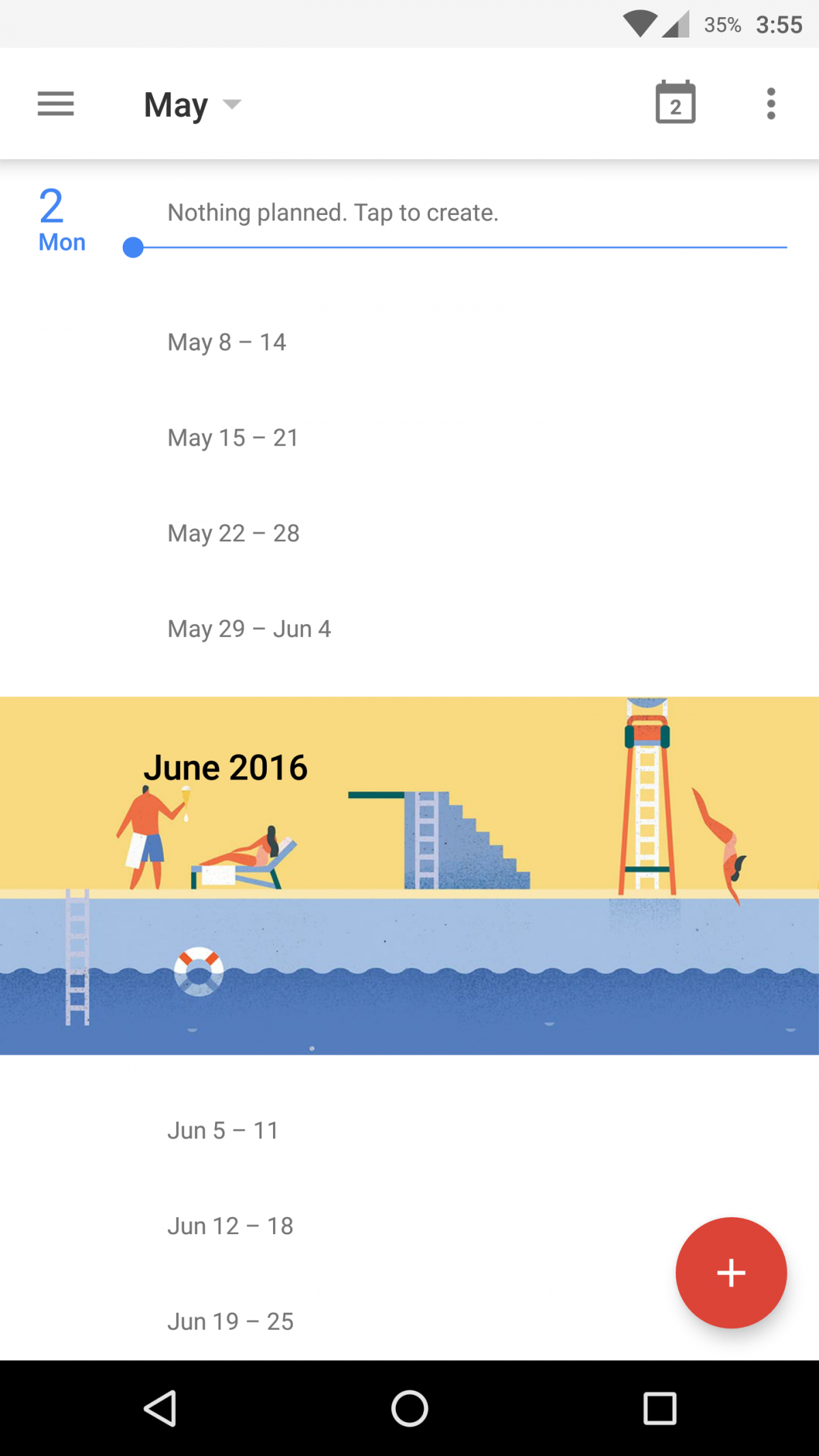In this image, set against a white background, we see a smartphone's screen displaying a planner app. 

Starting from the top left corner, there is a menu icon represented by three horizontal lines. To the right of this, the month "May" is displayed. On the top right corner, there's a calendar icon followed by an options icon indicated by three vertical dots. Just below the options icon, the date "Monday, May 2nd" is written in blue. Adjacent to this date is a prompt that reads, "Nothing planned, tap to create."

Below this notification, the calendar is segmented into weeks: May 8th to 14th, May 15th to 21st, May 22nd to 28th, and May 29th to June 4th. Under these dates, the header "June 2016" appears in black.

The background image features a vivid blue staircase leading to a swimming pool. The pool water is a dark blue. On the left of the pool is a staircase for climbing out. A distinctive visual feature is a person depicted sleeping on a bed next to the pool.

At the bottom of the image, subsequent weekly dates are listed: June 5th to 11th, June 12th to 18th, and June 19th to 25th. Finally, in the bottom right corner, a large red circle with a white plus sign inside serves as the "add event" button.

This detailed composition blends the functionality of a digital planner with the serene imagery of a swimming pool scene, seamlessly integrating usability with visual tranquility.